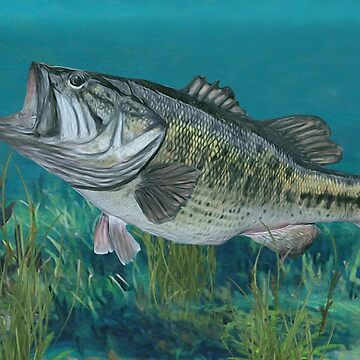The image depicts an underwater scene that appears to be a painting, likely done with oils. At the center of the image, there is a large fish shown from a side angle, its mouth wide open as if consuming krill. The fish is rendered in shades of gray, white, and features a striking gold streak that extends from its head to its tail. It is positioned diagonally and tilted upwards, creating a dynamic sense of movement as it heads towards the surface. The background is a gradient of blues, with lighter and darker shades indicating depth. Surrounding the fish, at the bottom of the image, are green and blue seaweed and various underwater plants. The whole composition is bathed in blue hues, giving an authentic underwater feel, with no text disrupting the serene aquatic landscape.